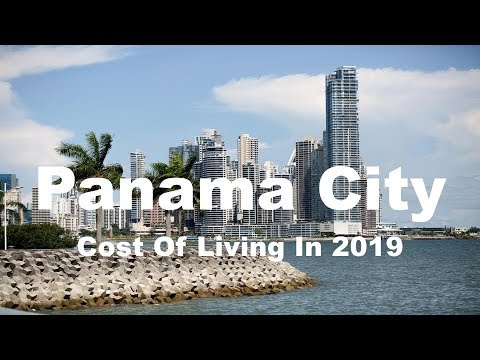A screenshot from the opening scene of a video, featuring a panoramic view of Panama City. The image is framed by black bars at the top and bottom, indicating a widescreen video format. The scene captures a serene coastal setting with a calm sea in the foreground, which includes a small island adorned with several palm trees. In the distance, a cluster of modern skyscrapers rises against a bright, sunny sky. Dominating the image, bold white text reads: "Panama City: Cost of Living in 2019," suggesting the video aims to provide information on the living expenses in Panama City during that year. There are no other textual elements or identifiers present to indicate the source of the content.